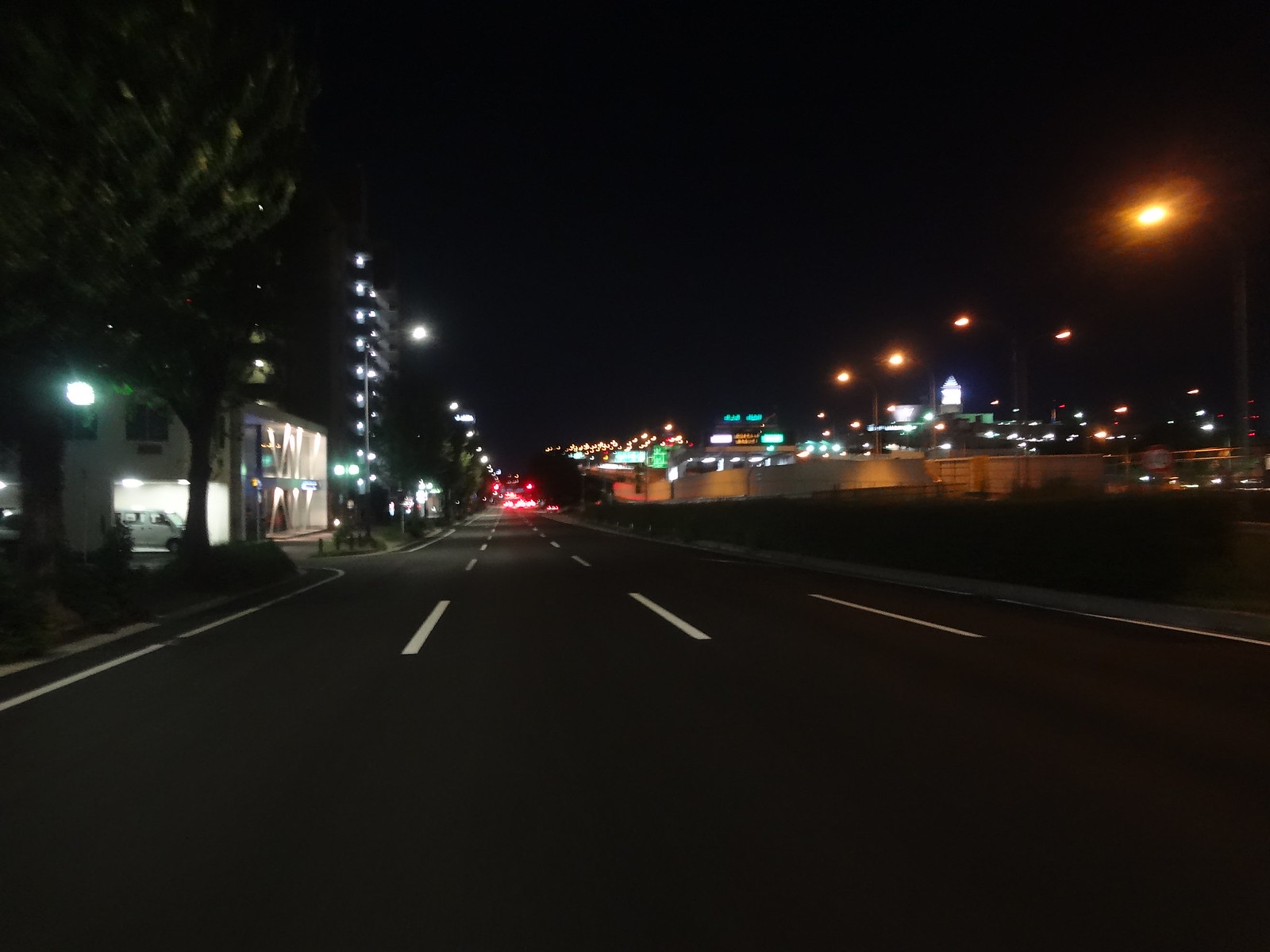This is an image of a nighttime urban highway scene taken from a large, square perspective. The background is predominantly black, with the top half of the image enveloped in the solid dark sky. The central part of the image features a four-lane road extending from the bottom towards the middle, marked by white dashed lines indicating the lanes. The road appears mostly black, blending with the night. On the left side, the road is flanked by buildings with illuminated signs and streetlights. There is a white van parked near a sidewalk lined with trees and more streetlights. Further down the sidewalk, additional trees can be seen. On the right side, a small grassy hill runs adjacent to the road, separating it from more distant buildings. The distant background reveals a scattering of city lights, including blurred signs on buildings and red taillights of cars, possibly waiting at a traffic light. These red lights appear tiny and indistinct due to the distance, adding to the depth and urban character of the scene.